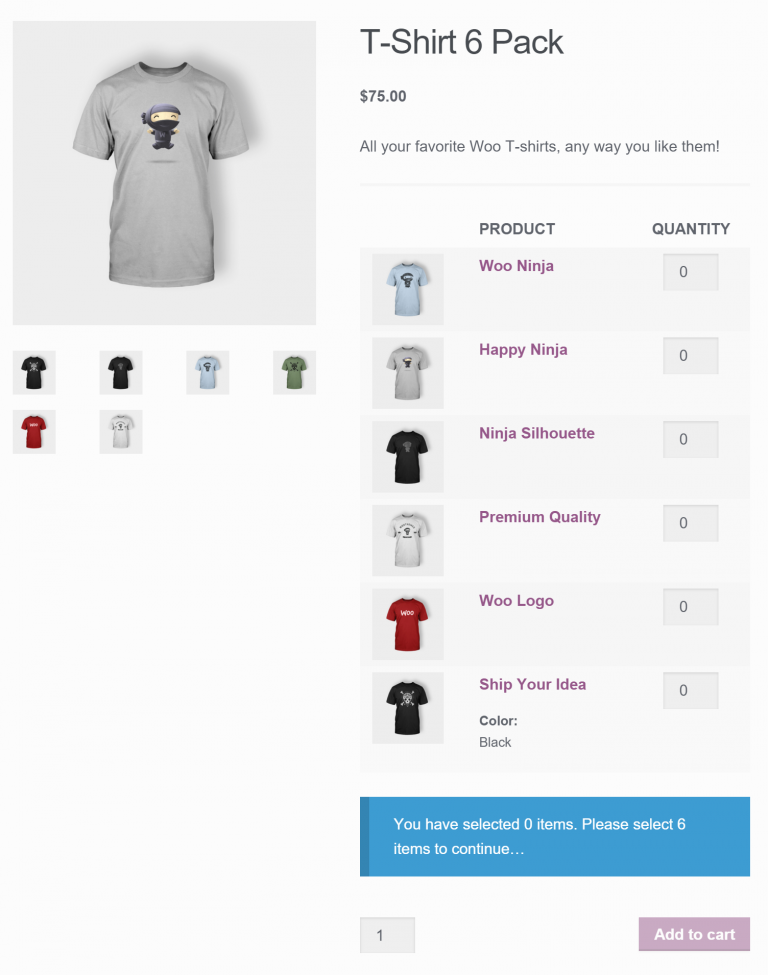A detailed product display showcases a six-pack t-shirt bundle for $75, featuring popular Woo-themed designs. Located on the right side, beneath a descriptive column, are the available t-shirt choices: "Woo Ninja," "Happy Ninja," "Ninja Silhouette," "Premium Quality," "Woo Logo," and "Ship Your Idea," all initially set at zero quantity. The text for product details is highlighted in pink, while the t-shirts appear prominently on the left side of the display. At the top left, a larger image displays the "Happy Ninja" t-shirt, featuring a solid gray color with a cheerful ninja graphic at its center. Below this main image, smaller thumbnails of the other designs are visible. A blue text box with white text instructs, "You have selected zero items. Please select six items to continue." Below this prompt, on the left-hand side, there is an "Add to Cart" button, styled in pink with white text.